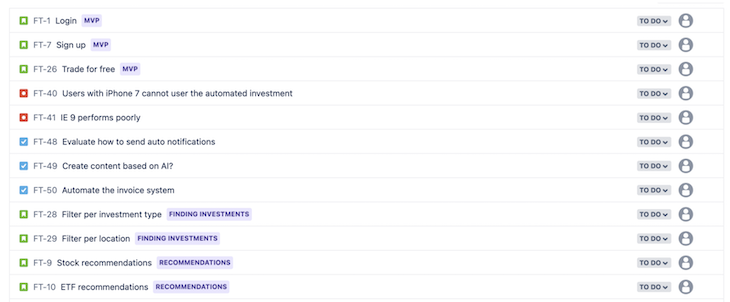This is a detailed descriptive caption:

The image is a screenshot of someone's to-do application displayed on a white background. The layout features multiple entries listed vertically, each corresponding to a task related to investment management. The first entry at the top left is labeled "FT-1 login" and is accompanied by the term "MVP" written in purple letters. On the far right of this entry, there is a to-do drop-down box followed by a small person icon.

Each entry on the to-do list follows a similar format, with a to-do drop-down box and a person icon to the right. The list includes tasks such as "FT-7 signup," "FT-26 trade for free," and "FT-40 users with iPhone 7 cannot use the automated investment." The nature of these tasks suggests that this is a to-do list for managing an investment portfolio. The very last entry is "FT-10 EFT recommendations," with "recommendations" noted in purple lettering to its right.

Overall, the to-do application appears structured and organized, enabling the user to efficiently manage various investment-related activities and troubleshooting tasks.